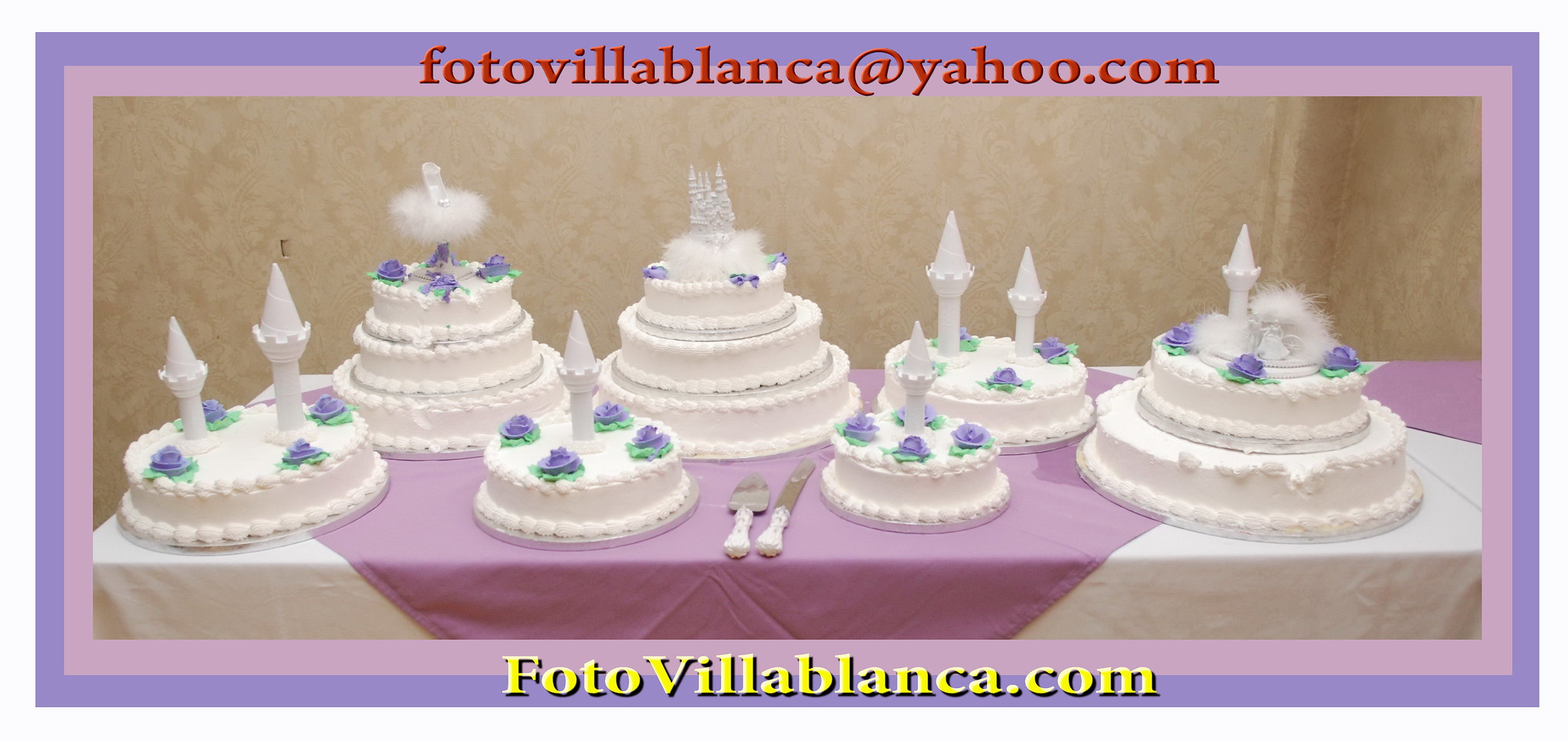This detailed photograph showcases an elaborate display of seven white wedding cakes adorned with intricate decorations. Each cake features purple flowers crafted from icing, accompanied by green leaves. The cakes are arranged on a long table draped with a white tablecloth, overlaid with a light purple-magenta cloth that is placed at an angle, creating a peak in the front.

The cakes include a mix of one-tier, two-tier, and three-tier designs:

- Four of the cakes are single-tiered, each topped with four purple flowers and green leaves. These cakes also display parts of castle towers as decorations, done in white.
  
- Among these single-tier cakes, there is one two-tier and two three-tier cakes. The two-tier and three-tier cakes also feature purple flowers and green leaves. Additionally, they showcase more complex white decorations resembling castle towers, trees, and other indistinct elements that seem furry, possibly representing fog or mist.

The backdrop of the image is a tan, sand-colored wall decorated with a floral design, enhancing the elegance of the scene. Framing the photograph is a double border: an outer light purple rectangle and an inner pink rectangle. The corners are neatly aligned with the edges of the table. 

Further details include two silver knives with white handles placed on the table. The photograph bears the contact information "foto Villa Blanca at yahoo.com" in red text at the top border and "foto Villa Blanca.com" in yellow text at the bottom border, completing the composition.